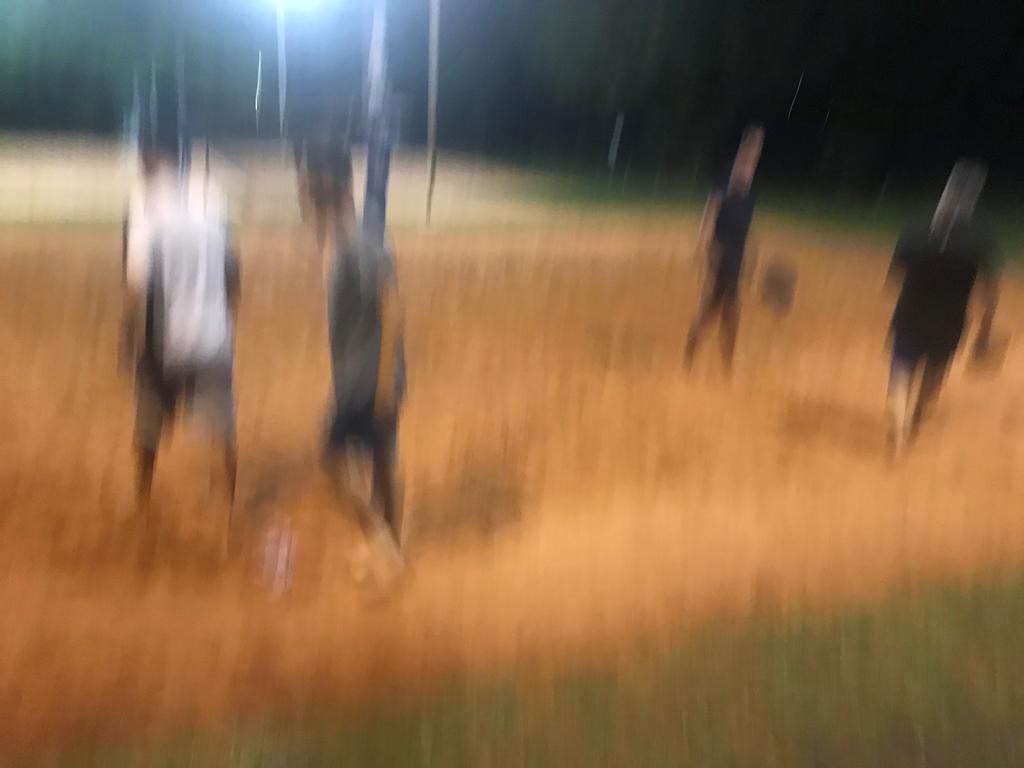The image depicts a nighttime scene with four people in an outdoor area adjacent to a basketball court, characterized by a brownish-orange dirt ground. Although the photo is notably blurry and distorted, it appears that the individuals, who are all wearing shorts, might be engaged in a game of soccer. Two men on the left are wearing white and gray shirts respectively, while the two on the right are dressed in black shirts. The presence of a ball on the ground suggests they are about to kick it. The scene is dimly lit by a nearby floodlight, and the dark background features some indistinct trees.